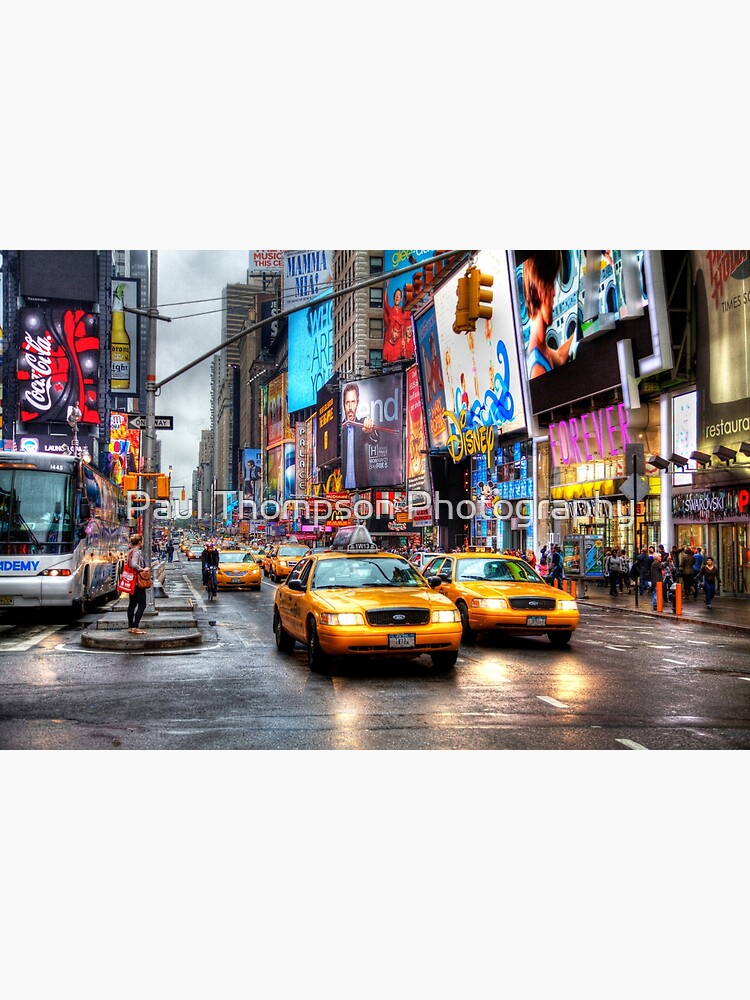The image captures a bustling city street scene, likely in the Times Square area of New York, just after a rainfall or during a drizzle. The cloudy, gray skies cast a moody ambiance, while the wet pavement reflects the glaring headlights of yellow taxi cabs visible from the front view, driving down a three-lane road. To the left, a city bus is parked alongside numerous pedestrians waiting at a crosswalk under an illuminated streetlight. More throngs of pedestrians bustle along the sidewalks, lined with an array of businesses ranging from small shops to towering skyscrapers. The landscape is vibrant with a multitude of neon signs and advertisements, including a prominent Coca-Cola sign and another likely from Mountain Dew. Additional notable storefronts include a Disney store and perhaps a Forever 21. Colorful reflections and signage add lively pops of black, red, white, blue, and yellow to the busy streetscape. Overhead, a yellow traffic light hangs from a pole, and across the center of the image lies a watermark: Paul Thompson Photography.